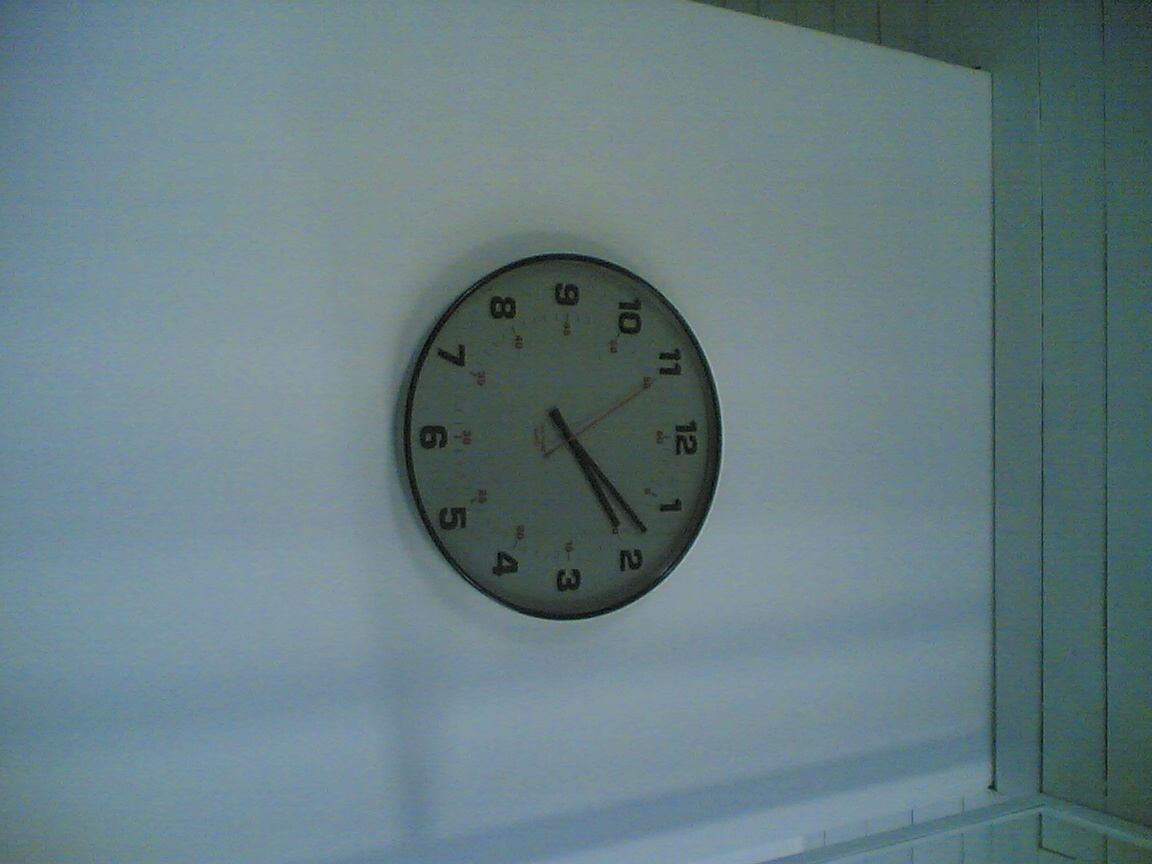A stylish interior scene features a juxtaposition of two walls: a light gray wall on the left and a slightly darker gray wooden wall on the right. At the center of the light gray wall hangs a prominent round clock with a black frame and a white face, accented by regular black numerals and hands. Intriguingly, the clock is oriented sideways, positioning the 9 and 3 where the 12 and 6 usually reside, and vice versa. The composition includes reflections of windows in the background, adding depth and a sense of natural lighting, with a distinct shadow cast by the clock providing subtle texture to the scene.